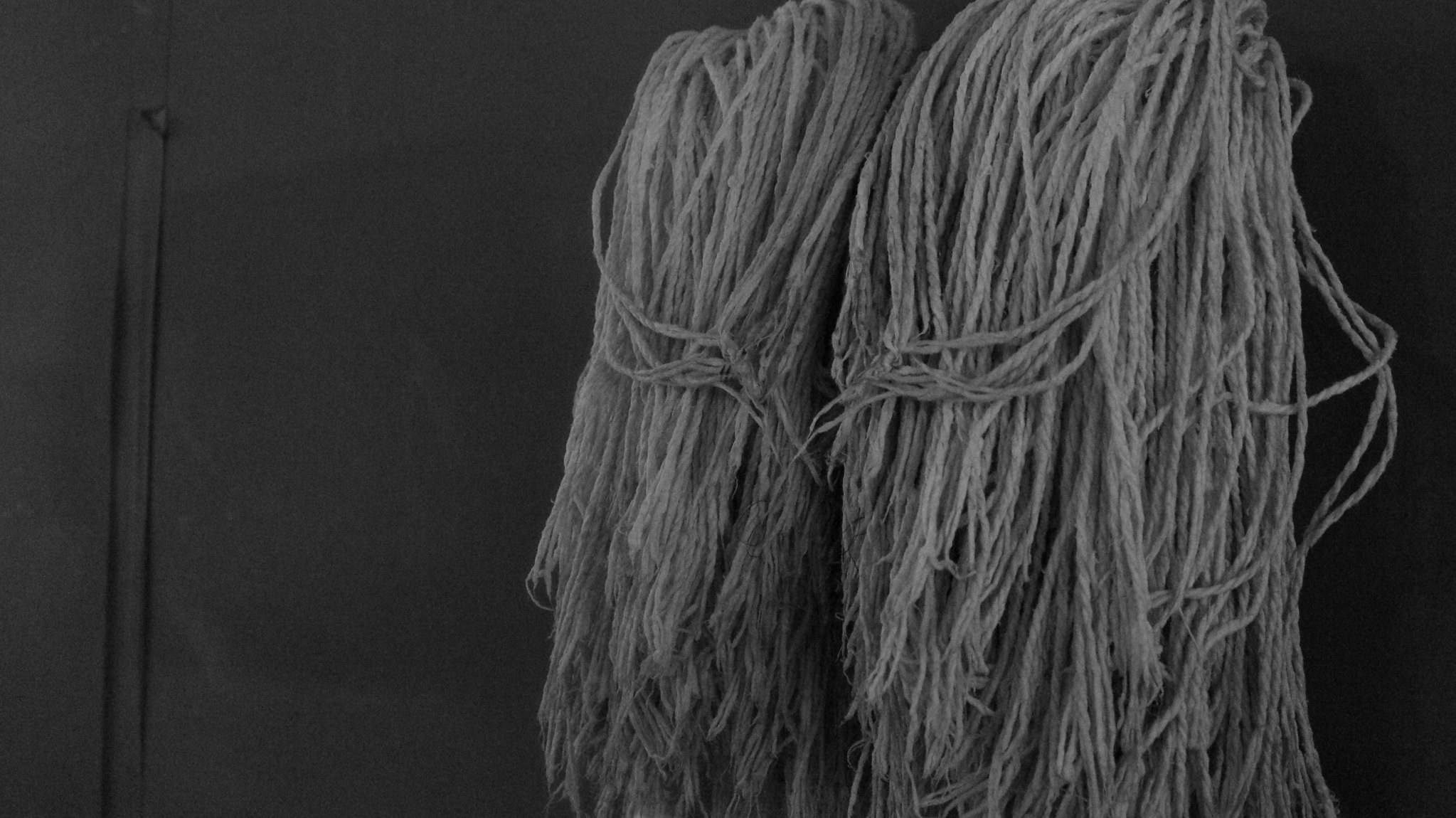The image features a close-up of two large, traditional string mop heads, characterized by their thick, grayish-white yarn strands. The photograph appears to be in black and white, set against a solid, dark gray background that might be a wall or even a mirror. The scene is lit in such a way that the mop heads, especially their individual yarn threads, are distinctly visible and appear quite full and robust. A mop stick is partly visible in the lower left corner of the image, emerging from one of the mop heads. A vertical seam or line on the left side of the background subtly accentuates the division between the two mop heads, giving the composition a slightly mirrored effect. Overall, the photograph's stark contrast highlights the texture and volume of the worn mop heads, drawing attention to their industrial utility.